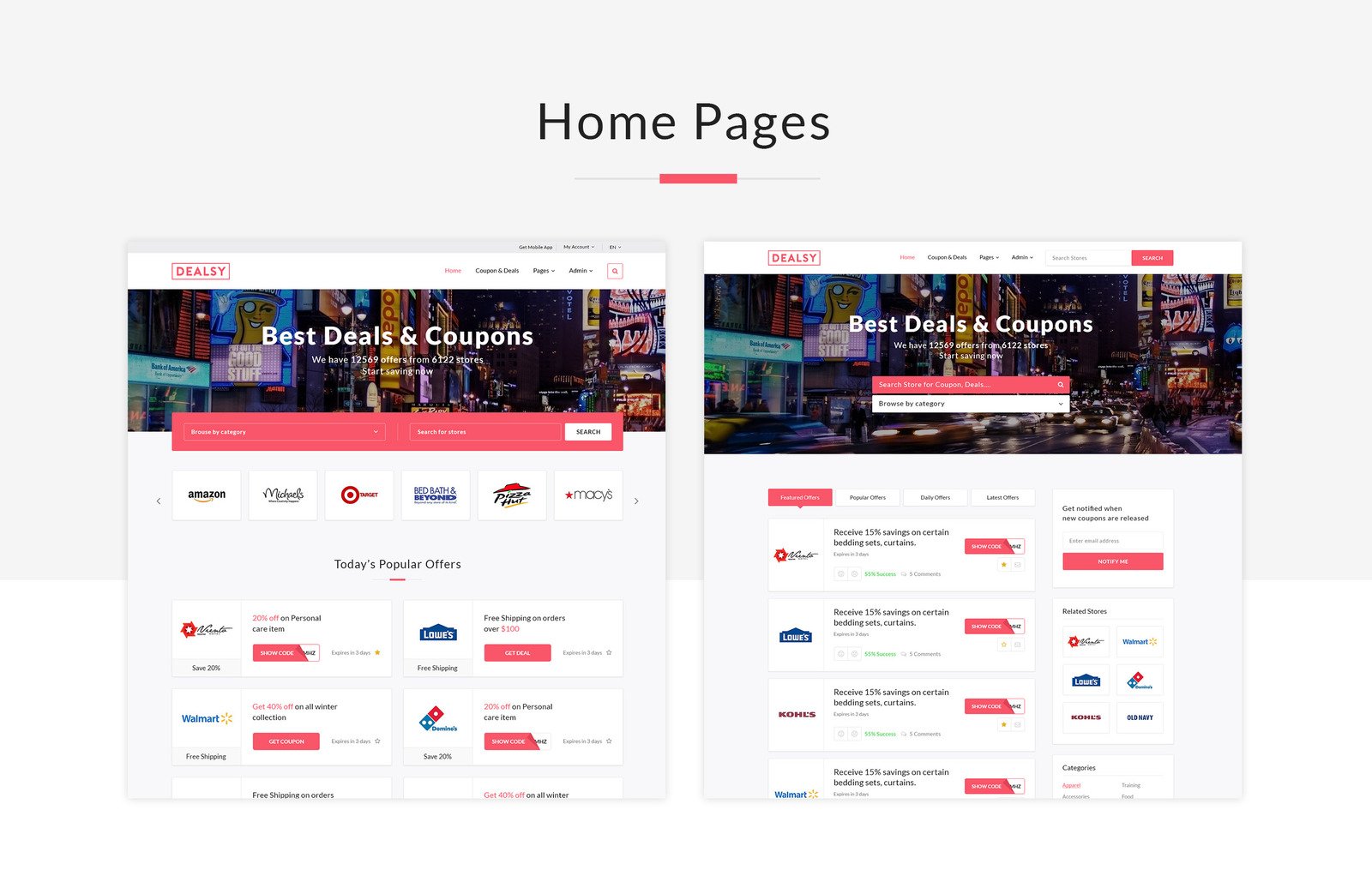The image presents a comparison of two potential homepages for the website DealZ. The background of the image is a gradient, with the top two-thirds in a silvery gray hue and the bottom third in white. At the top center, the text "Home Pages" is prominently displayed in black, underlined by a thin gray line. A thicker red line intersects this underline at the center, adding a splash of color.

Beneath this header sits a screenshot comparison of two homepages from DealZ. Both homepages feature a consistent white bar at the very top, containing the website's name "DealZ" in red text within a red rectangle. Just under this, both have a menu bar, though it's too small to discern the exact options. The main visual of both homepages includes a busy shopping district background image with the phrase "Best Deals & Coupons" emblazoned in white text. On the left homepage, this text is larger and more readable compared to the right homepage, where it is smaller.

Below these elements, the homepage on the left includes a search bar in a bold red with a white search button situated beneath the background photo, while the right homepage has the search bar integrated directly onto the image.

Descending further, the left homepage showcases a horizontal, scrollable section with left and right navigation arrows displaying logos of various retailers. Visible among them are Amazon, a partially obscured "M" retailer (likely Michaels), Target, Bed Bath & Beyond, Pizza Hut, and Macy's. Directly beneath this are larger white boxes labeled "Today's Popular Offers" featuring deals from Lowe's, Walmart, and Domino's Pizza.

Conversely, the right homepage lacks the horizontal scrolling feature for retailer logos but retains the larger white rectangles highlighting similar special offers from Lowe's, Walmart, and other retailers.

This image effectively contrasts the design elements and layout differences between two proposed DealZ homepages, emphasizing variations in readability, search bar placement, and display of retailer options.